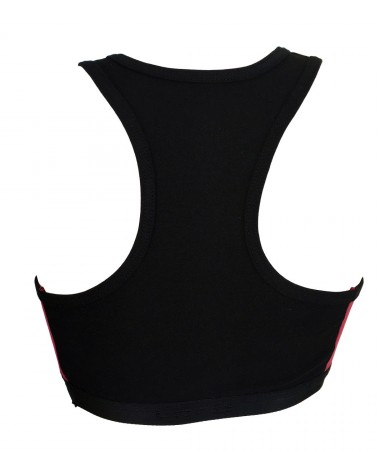The image features a solid black object against a stark white background, capturing a shapely, curved form that immediately draws the eye. This intriguing black shape, free from any visible dates, times, or locations, stands alone without any people or animals in the frame. With no additional objects, the focus remains solely on this form, characterized by its distinct silhouette. 

The shape resembles that of a woman’s halter top or possibly the chest protector worn by a baseball catcher, featuring a high collar that extends up to the neck before flaring out towards the sides and tapering into a narrow lower portion resembling a waistline. This gives it the appearance of a dress or a piece of sportswear, yet it remains ambiguous due to the lack of quilting or padding, often characteristic of a catcher’s gear, and the absence of any supporting mannequin or display. The overall presentation is simplistic yet captivating, defined by its clean, flowing lines and a striking contrast between the black shape and its white background.